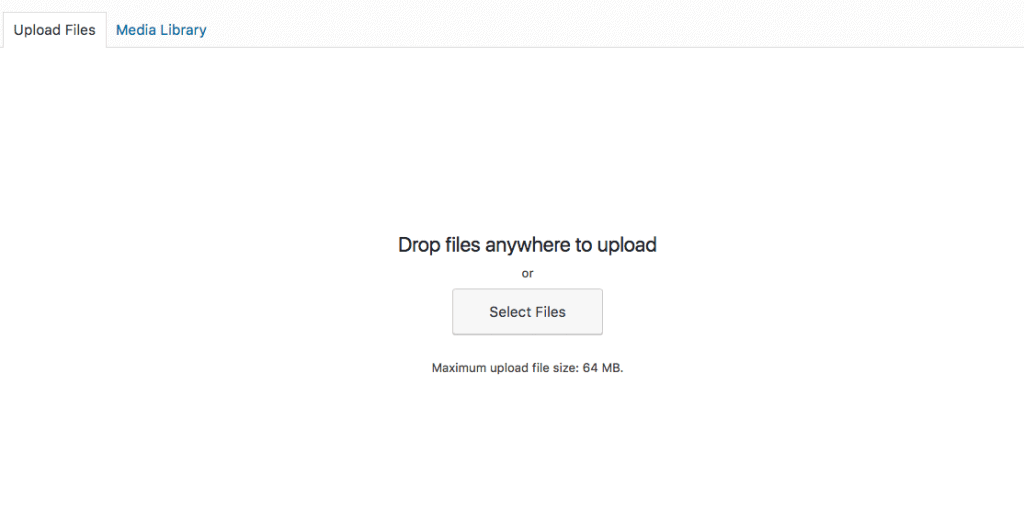The image displays a user interface from an application featuring multiple selectable tabs. The currently active tab, labeled "Upload Files" with both "U" and "F" in uppercase, is highlighted in black text on a white background. The tab's content prominently features a larger font message in the center: "Drop Files Anywhere to Upload." Below this, the word "OR" is written, followed by a light grey button with the label "Select Files." Beneath the button, a reminder states that the maximum upload file size is 64 megabytes. This screen clearly provides options for users to either drag and drop a file or click the "Select Files" button to browse and choose a file for uploading.

Adjacent to the active tab is another tab labeled "Media Library," which is not selected and is displayed in blue text. Both tabs are set against a very light grey banner that runs horizontally across the top of the image, underscoring the "Upload Files" tab as the current selection.